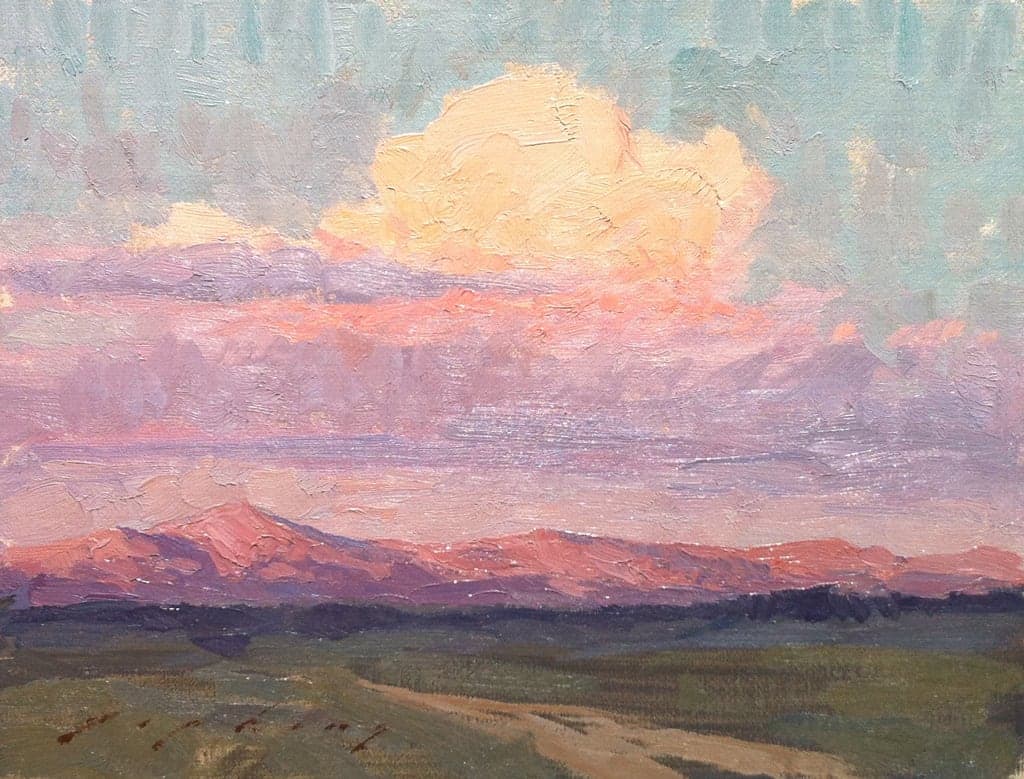The painting is a large, square watercolor work depicting a landscape that appears to be inspired by the Great Plains of the United States. The composition is divided into several distinct sections, each characterized by its own color and form. At the top of the painting, a sky that transitions from a gradient of purple, pink, and yellow to a more standard light blue dominates the scene. A large, yellowish-white cloud is prominently centered in this sky. 

Below the sky, the middle section features an outline of mountains, blending pink and brownish-gray hues, possibly indicating the effect of fading light. These mountains present a more detailed outline, particularly towards the bottom where they appear predominantly brown. 

The bottom section of the painting showcases green fields with rocky and light brown elements. A distinctive dirt path painted in brown cuts diagonally through this green expanse. Towards the lower left corner, several brown smears suggest the presence of animals. Overall, the painting, while abstract in its execution, effectively conveys a sense of natural landscape with its vibrant use of colors and forms.